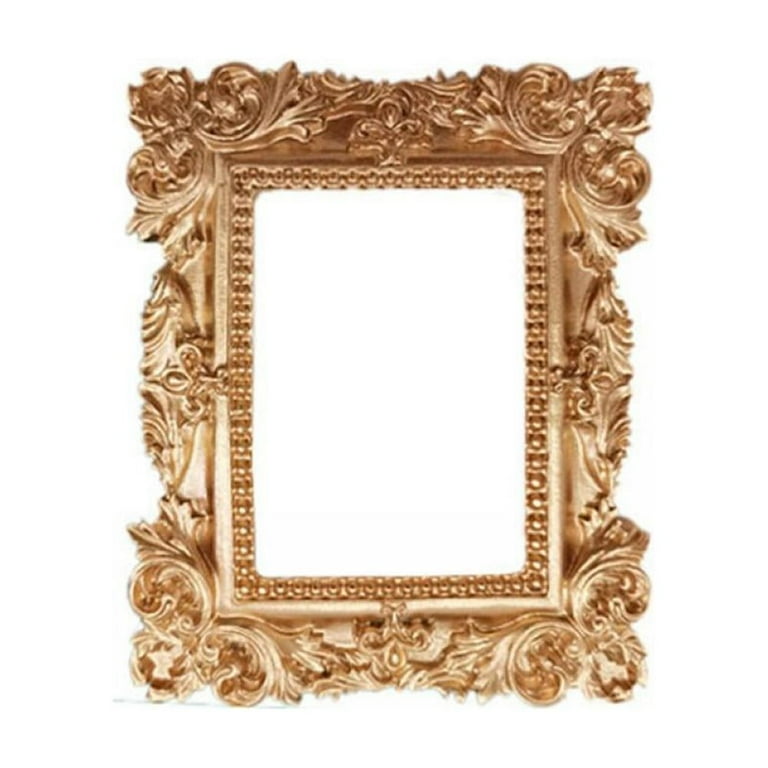The image depicts an elaborately designed, gold-colored picture frame set against a clean, white background, possibly taken in a lightbox. The frame is centrally positioned and features a highly ornate pattern, characterized by symmetrical filigree with floral motifs at the corners and extending leaves or branches toward the center. The craftsmanship appears intricate, with the possibility of it being carved wood or a detailed computer-generated design. The frame is notably thick and wide, creating a striking contrast with the empty space it encloses. The photograph itself appears somewhat pixelated and blurry, giving it a less polished, product-photo-like quality.